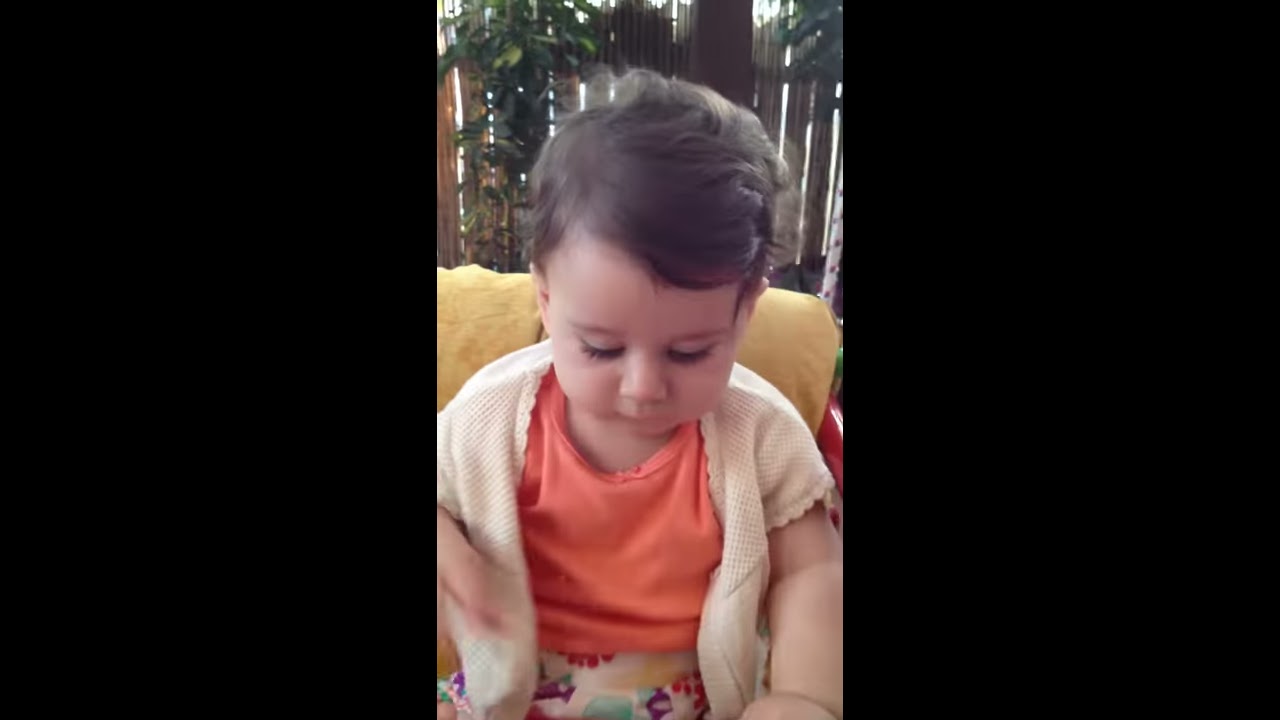The photograph captures a young toddler, possibly around three or four years old, seated against a dull yellow cushion with a wooden fence serving as the backdrop. The child, who appears to be Caucasian with short dark brown hair and thick, long eyelashes, is intently looking down at something they are holding with their left hand. They are dressed in a short-sleeved orange t-shirt layered under a light beige short-sleeved sweater. The bottoms feature a colorful print with various designs in yellow, red, light blue, and purple. Notably, the child's right hand is in motion, resulting in a blurry effect. Behind the child, sunlight filters through the wooden fence, which is partially adorned with climbing plants.